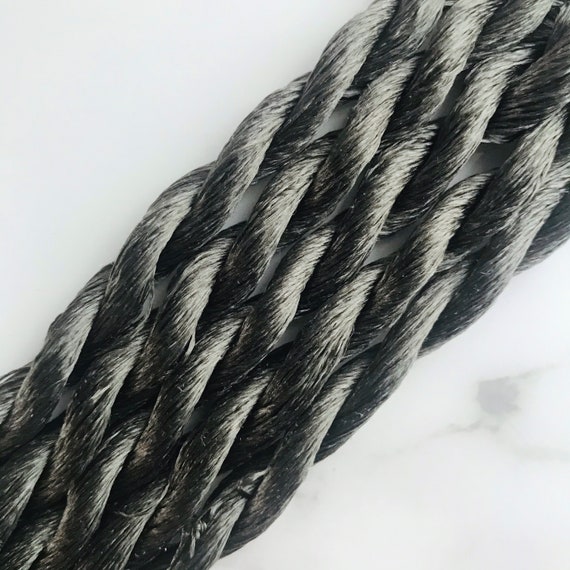This black and white square image features an extreme close-up of a thick, tightly woven braid, which could be either human hair or a rope made of twine or burlap. The braid, composed of at least five intertwining strands, spans diagonally from the top right to the bottom left corner against a blurred, white background. Notably, there is a small dot or smear beneath the bottom half of the braid on the right side. The photo captures the intricate weaving pattern and some fraying at the bottom, emphasizing the fibrous texture and highlighting the serpentine flow of the strands.